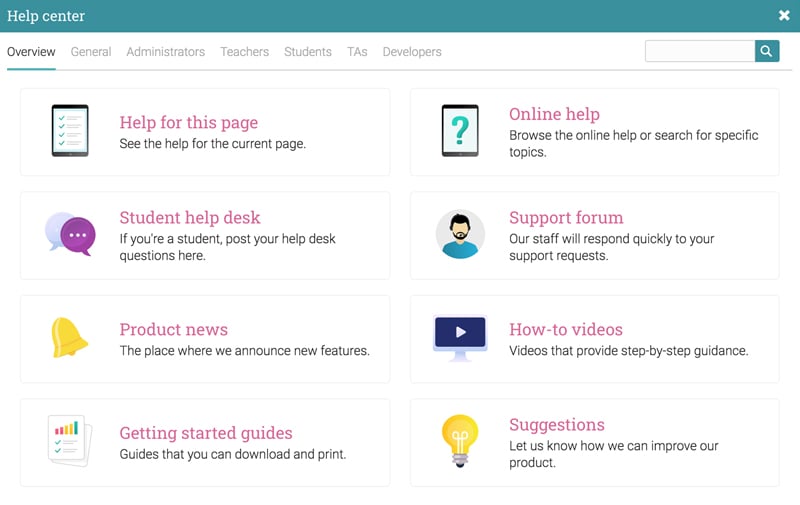The image features a clean white background, dominated by a blue header box at the top, which is labeled “Help Center.” To the right of this header, there is an "X" icon, presumably to close the Help Center interface.

Below the header, user navigation options are listed in a horizontal menu. The "Overview" tab is underlined, indicating it is currently selected. Other menu options include "General," "Administrators," "Teachers," "Students," "TAs," and "Developers."

Beneath the menu, there's a search box allowing users to find specific help topics. Below the search box is a dividing line sectioning off the navigation area from the help topic listings.

The listed help topics are divided into two main groups, each with its items highlighted in pink. The first group includes:
- Student Help Desk: For students to post their help desk questions.
- Product News: Announcements about new features.
- Getting Started Guide: Guides that can be downloaded and printed.

The second group includes:
- Online Help: To browse help topics or search for specific information.
- Support Forum: A place where staff will quickly respond to support requests.
- How-To Videos: Videos offering step-by-step instructions.
- Suggestions: A section for users to provide feedback on how to improve the product.